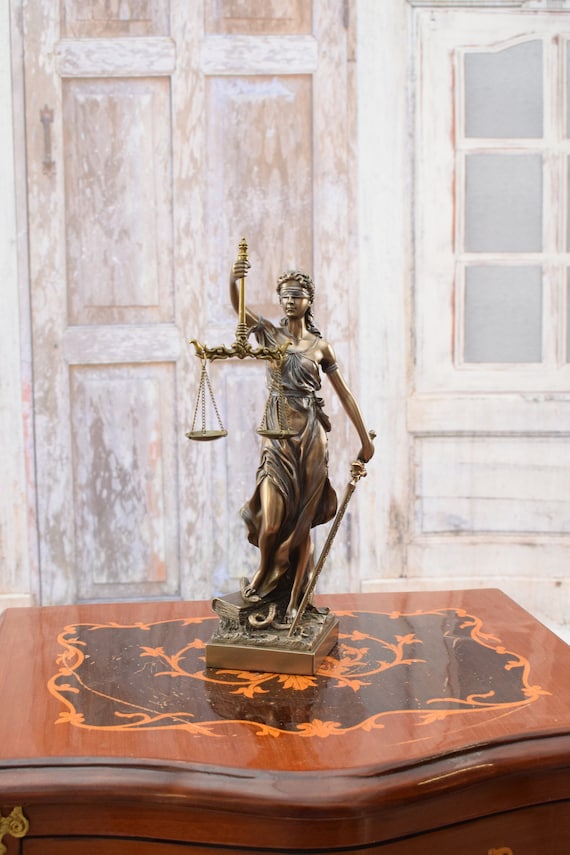In this color photograph with a portrait orientation, a bronze statue of a young woman stands prominently on a detailed wooden desk. The dark brown desk with a light brown inlaid top features an intricate design of vines, flowers, and leaves, outlined in gold. The woman, embodying the classical figure of Lady Justice, holds a pair of scales in her raised right hand and a sword pointing downward in her left hand. She is blindfolded, wears a long, flowing robe, and a corona of flowers and leaves adorns her head. At her feet, a snake is coiled, adding a mythical dimension to the piece. The desk is positioned in front of a distressed, white-painted door with visible wood beneath the chipped paint, contributing to a rustic backdrop. The cabinet on the right is also white, complementing the overall vintage aesthetic of the scene. The statue's realistic and representational style captures meticulous details, evoking classical Greek or Roman influences.